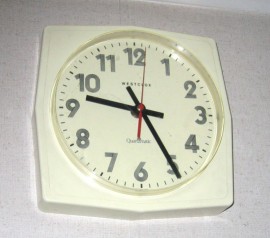This is a detailed image of a wall clock hanging on a gray, possibly wallpapered wall. The clock itself is a square with off-white, cream-colored edges featuring pointed accents at the 12, 3, 6, and 9 positions. Its face is similarly off-white, contrasting with the black minute and hour hands. The time displayed is 9:25, and a red second hand is positioned precisely between the 1 and 2-second marks. A light source illuminates areas around the numbers 1 and 7, creating subtle shadows moving toward the upper left corner of the image.